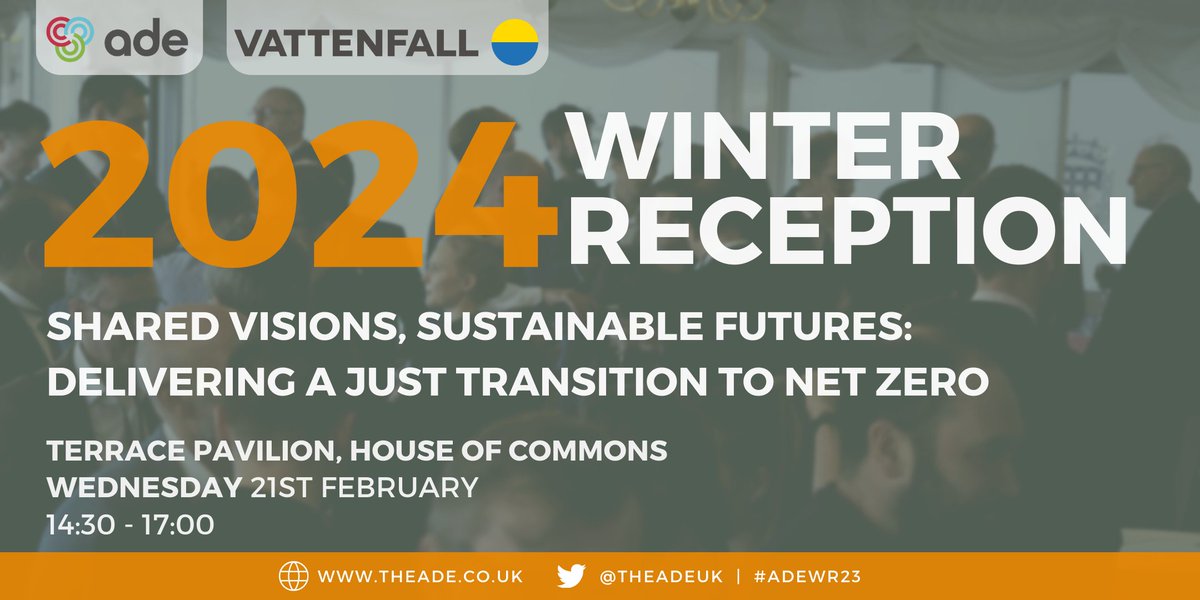This image is a detailed, digitally created poster advertising the 2024 Winter Reception event. It features a grayed-out background image of a group of indistinct people in a conference room, creating a professional atmosphere. Dominating the center of the poster, “2024” is displayed in bold orange print, with “Winter Reception” written beneath it in bold white letters. Below this, in smaller white print, it reads, “Shared Vision Sustainable Futures Delivering a Just Transition to Net Zero.” 

Further down, an additional line of small white text specifies the event details: “Terrace Pavilion, House of Commons, Wednesday, 21st February, 1430-1700.” 

In the upper left corner, there are two gray beveled rectangles. The first has interlinked circles colored blue, green, and red with the gray text “ADE” beside them. The second rectangle has the text “Vattenfall” beside a circle split into a yellow top half and a blue bottom half. Below these rectangles, “2024” is repeated in bold orange text.

Running across the bottom of the poster is an orange footer stretching the width of the image. At its center-left, it features a small white globe icon followed by the URL “www.theade.co.uk” in white print. To the right, a white bird icon and the handle “@theadeuk” are positioned next to a vertical line, followed by the hashtag “#ADEWR23.”

The overall color scheme of the poster includes shades of gray, with accent colors of orange, white, yellow, blue, red, green, and black, emphasizing the key information in a visually appealing manner.